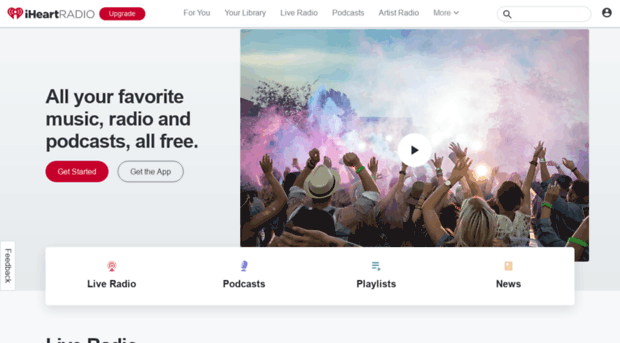This image showcases the iHeartRadio interface in detail. On the left side, the red iHeartRadio logo is prominently displayed, with clickable options adjacent to it including: "For You," "Your Library," "Live Radio," "Podcasts," "Artist Radio," and more. A search bar is situated below these options, providing easy navigation. Further down, the categories "Live Radio," "Podcasts," "Playlists," and "News" are listed. Dominating the center of the screen is a bold headline declaring, "All your favorite music, radio, and podcasts all free," accompanied by clickable buttons for "Get Started" or "Get the App." To the right, an eye-catching photo depicts a large crowd of people, reminiscent of Burning Man, with their arms raised in celebration against a backdrop of sky and overgrown bushes. The scene is vibrant with pink, blue, and purple smoke, creating a dynamic and colorful atmosphere. At the center of the image is a white dot with a black arrow, indicating a clickable video link. The smoke displays impressive gradients and shades, including muted tones of purple to pink and gray.